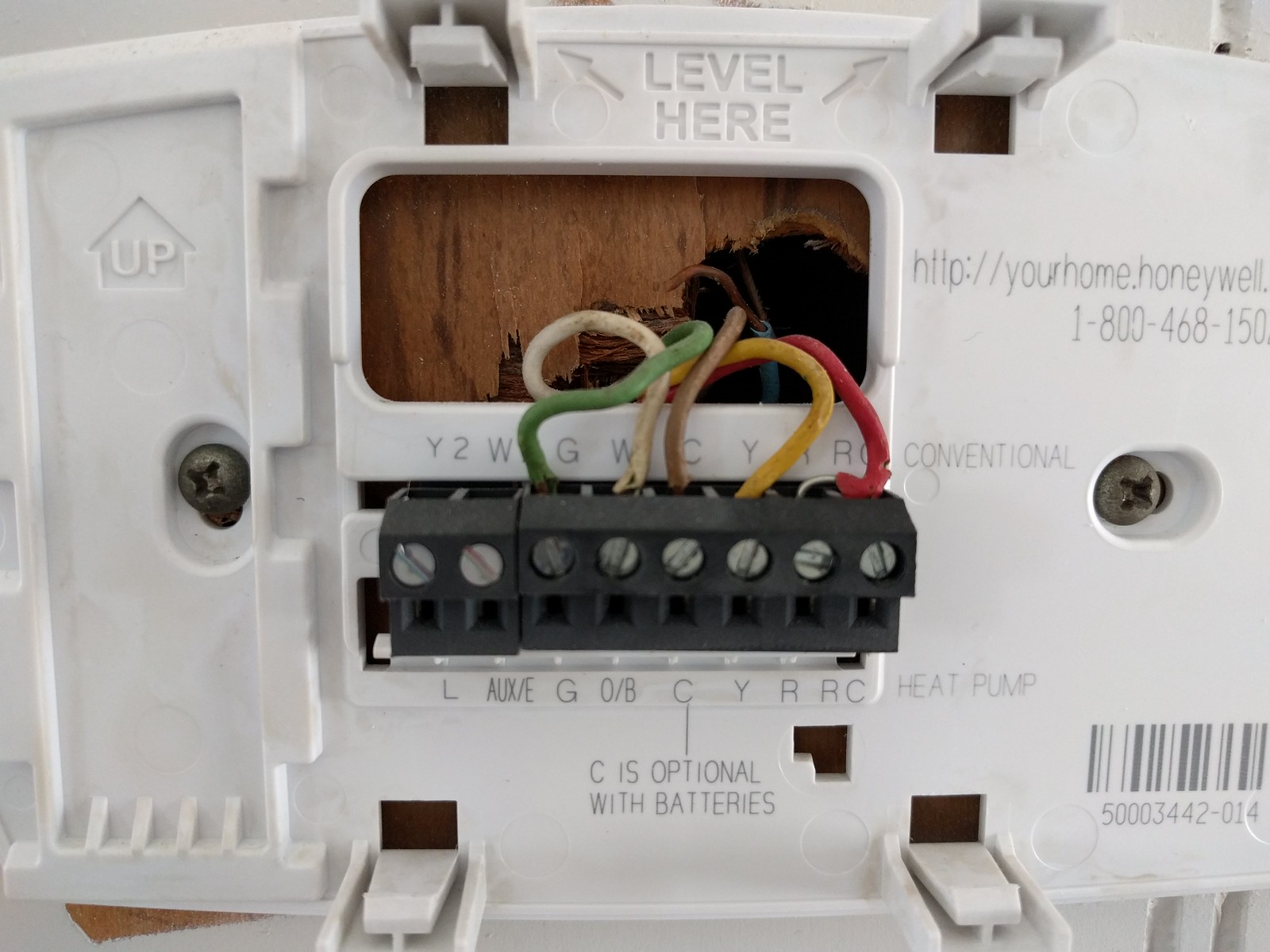This landscape-oriented photograph captures a close-up view of the bottom section of an electrical unit encased in plastic. Central to the image are various colored wires—green, cream, brown, yellow, and red—emerging from a hole in a wooden panel-like structure. Each wire is meticulously connected to a black connector using silver nails, with each nail corresponding to specific labels above: Y, 2, W, G, W, C, Y, I, and R. These labels likely indicate the wiring connections for the electrical components. The plastic casing of the unit envelops these connections, hinting at a sophisticated and organized electrical system.